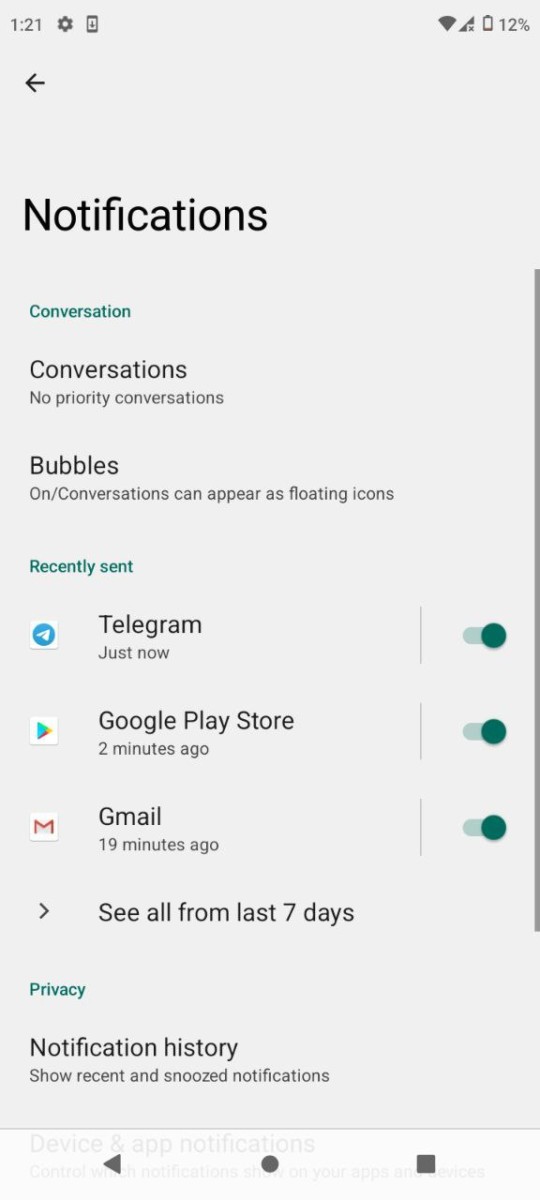Screenshot of a Cell Phone Notification Settings Page

The screenshot captures the notification settings page of a cell phone. It is 1:21 PM, indicated at the top of the screen. Adjacent to the time, there is a settings icon and a phone updates icon. On the right-hand side of the status bar, a Wi-Fi icon is visible alongside an icon indicating no cell phone signal. The battery is critically low, showing a charge of only 12%.

Below the status bar, there is a left-pointing arrow, functioning as a back button. Underneath this arrow, the word "Notifications" is displayed in black text, followed by "Conversations" in green text. Further down, the word "Conversations" appears again in black text, with the phrase "No priority conversation" written in gray.

The next section is labeled "Bubbles," with the explanatory text "On / Conversations can appear as floating icons" in gray. Below, the section titled "Recently sent" is highlighted in green letters. It lists recent notifications: "Telegram" with a "Just now" time stamp, "Google Play Store" with a "2 minutes ago" time stamp, and "Gmail" with a "19 minutes ago" time stamp. To the right of each of these items are green toggle buttons, all of which are turned on.

At the bottom of the page, a dropdown menu arrow provides the option to "See all from the last 7 days," followed by the word "Privacy" in green text.